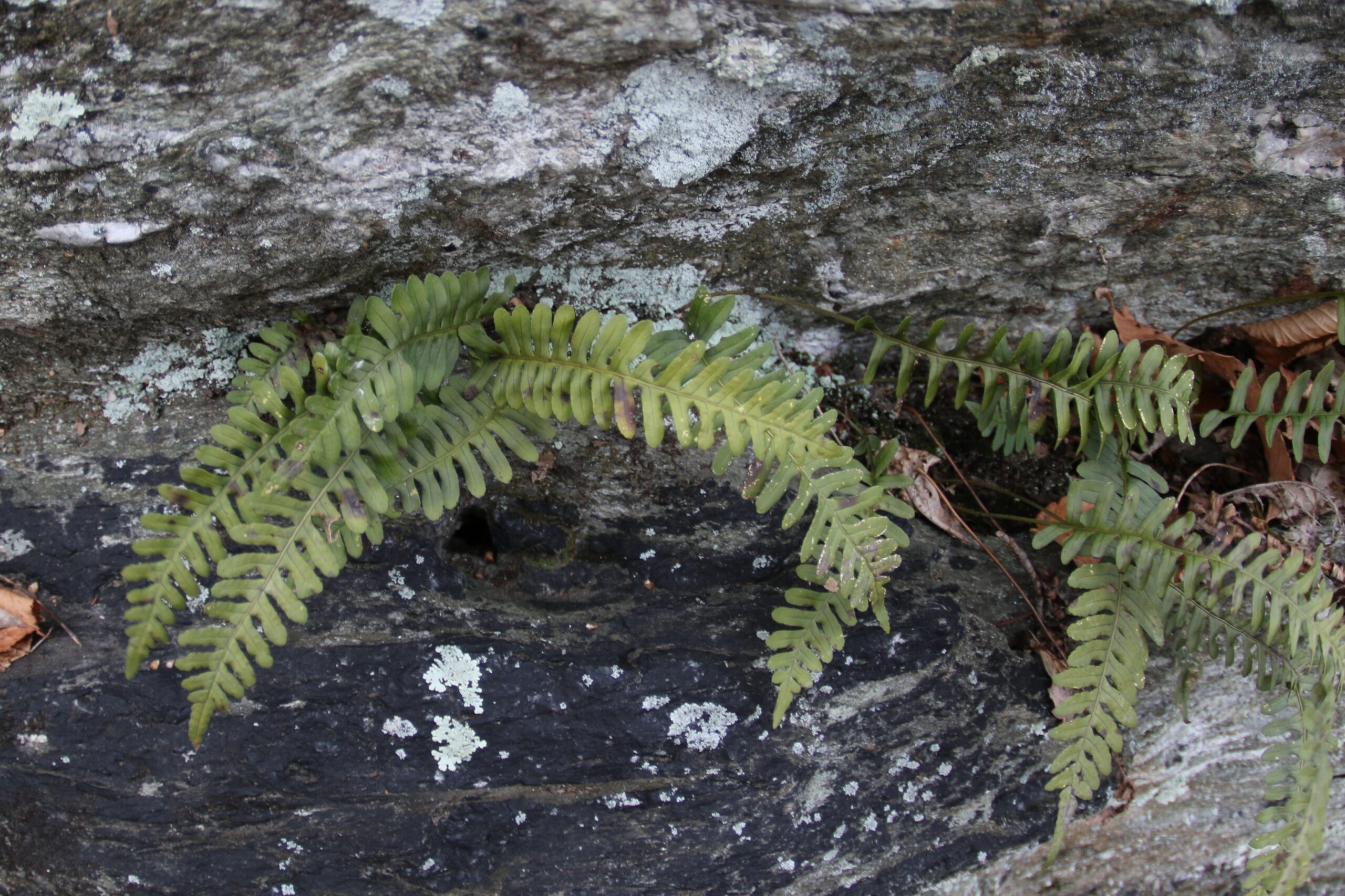This color photograph captures a close-up view of a rocky landscape where resilient plants, possibly ferns, grow in the crevices. The scene features a striking contrast between two main rocks - the bottom one is a deep black while the top rock is a light gray. Scattered across these rocks are patches of very light green lichen, more profuse on the top rock and more sparse on the bottom one. Amidst these rocks, especially in the crack between the dark and light colored stones, several plants with light green oval leaves sprout directly from the central stem without separate leaf stems. The leaves emerge predominantly in the center and towards the right side of the photo. Among these living plants, there are dead, dried leaves and visible soil, mostly concentrated on the right side. Additionally, a dried leaf can be spotted lying on the left-hand side of the image.